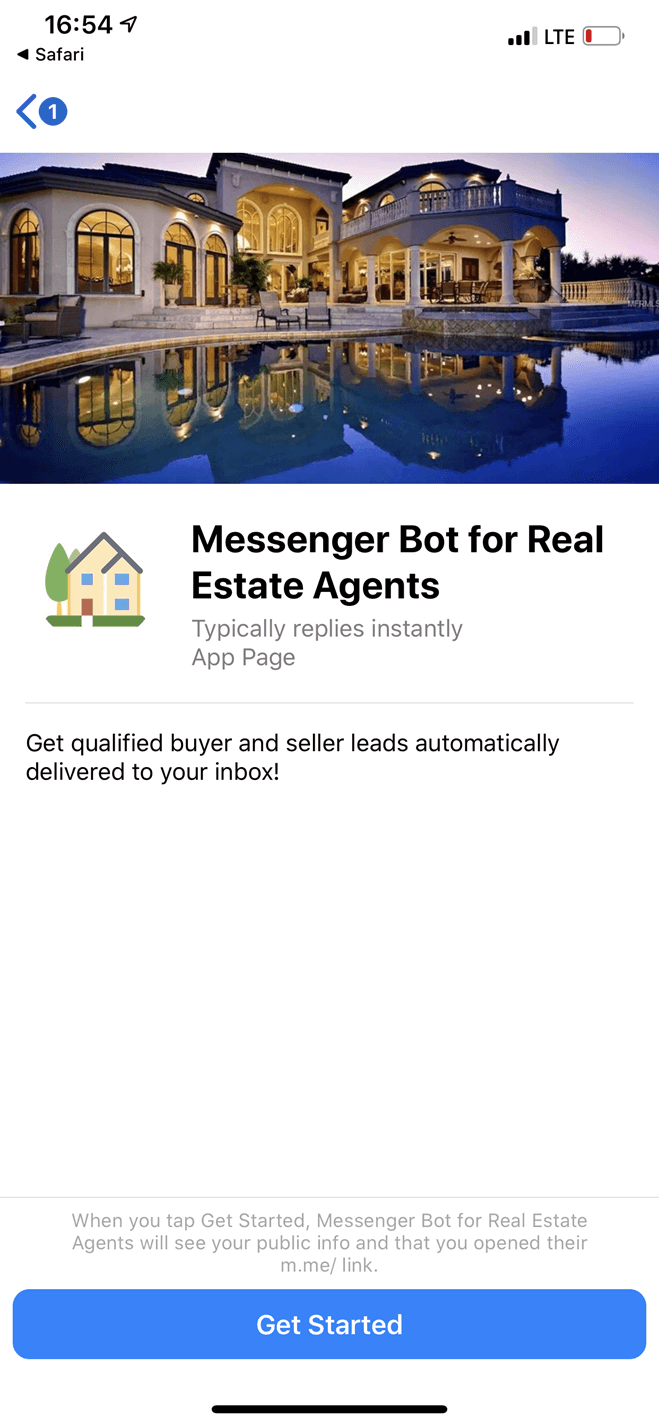In the screenshot of a mobile device, situated at the top right corner, the network signal icon displays 3 out of 4 bars with an 'E' indicating an EDGE connection. Adjacent to it, the battery icon is entirely empty, suggesting the device needs charging immediately. The current device time, displayed at the top left, reads 4:54 PM.

Below this status bar, the screen shows the Safari browser open with a webpage loaded. The main content of the page is a promotional banner for a messenger bot designed specifically for real estate agents. This bot is advertised to help generate qualified buyer and seller leads, which are automatically delivered to the agent’s inbox. The banner prompts the user to tap 'Get Started' to use the messenger bot.

Upon tapping 'Get Started,' a message appears indicating that the messenger bot will access the user's public information. The webpage appears to be from a domain resembling "dot e open jar main dot main link." Additionally, there is an image of a building within the promotional content, reinforcing the real estate theme of the banner.